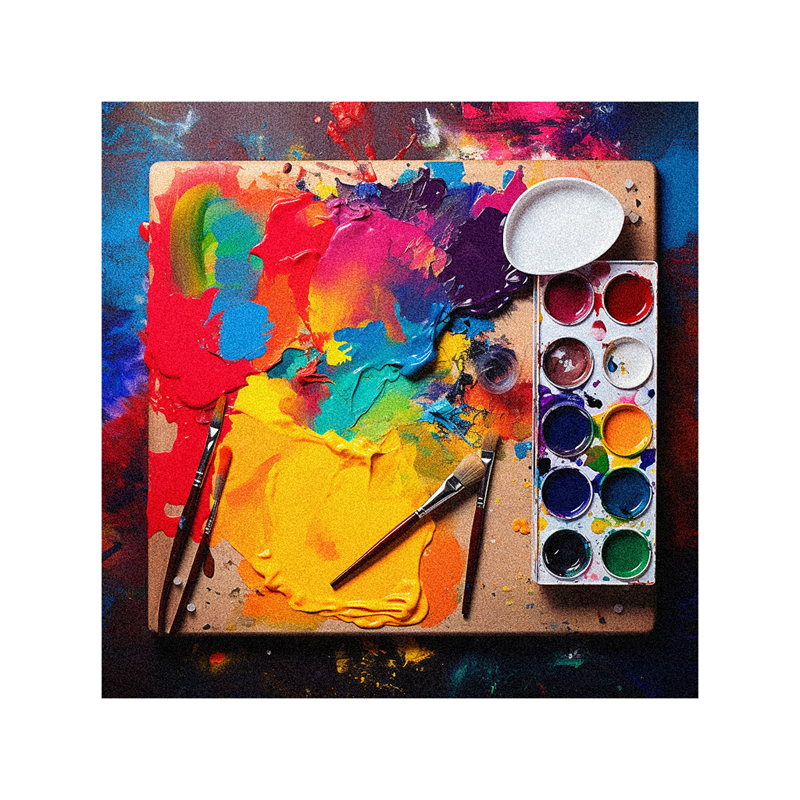In this photograph, an artist's workspace is meticulously captured, showcasing a makeshift palette atop what appears to be a cork or wooden board with various paint splotches, reminiscent of a colorful, painted drawing. To the right, there is a set of paints featuring a vibrant array of colors including yellows, blues, reds, purples, greens, whites, blacks, and oranges. Beside the paints lies a somewhat crumpled, likely water cup, presumably used for mixing. Scattered on this artistic setup are four paintbrushes of varying sizes and a multitude of thickly mixed oils or acrylics, vividly reflecting the creative and dynamic atmosphere of the space. The board, possibly used by the artist to hold or mix paintings, is vibrant and diverse in its colors and textures, underscoring the artistic flair of its user.